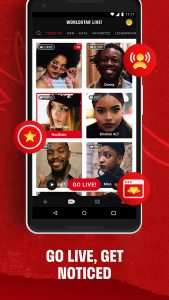The image showcases a mock-up of an Android phone, prominently displaying a live-streaming screen. The phone is set against a vibrant red background, with the text "World Star Live" emblazoned at the top, signifying a service from World Star Hip Hop. On the phone's screen, six young Black musical artists—four women and two men—are featured, each appearing poised and attractive. Though the surrounding text is blurry and unreadable, the phrase "Go Live, Get Noticed" is clearly visible, implying an opportunity for these aspiring artists to gain exposure and potentially attract talent scouts. The phone itself is sleek and predominantly black, accentuated with silvery bezel details. The rest of the image uses a dark background with contrasting white text to highlight other site elements.